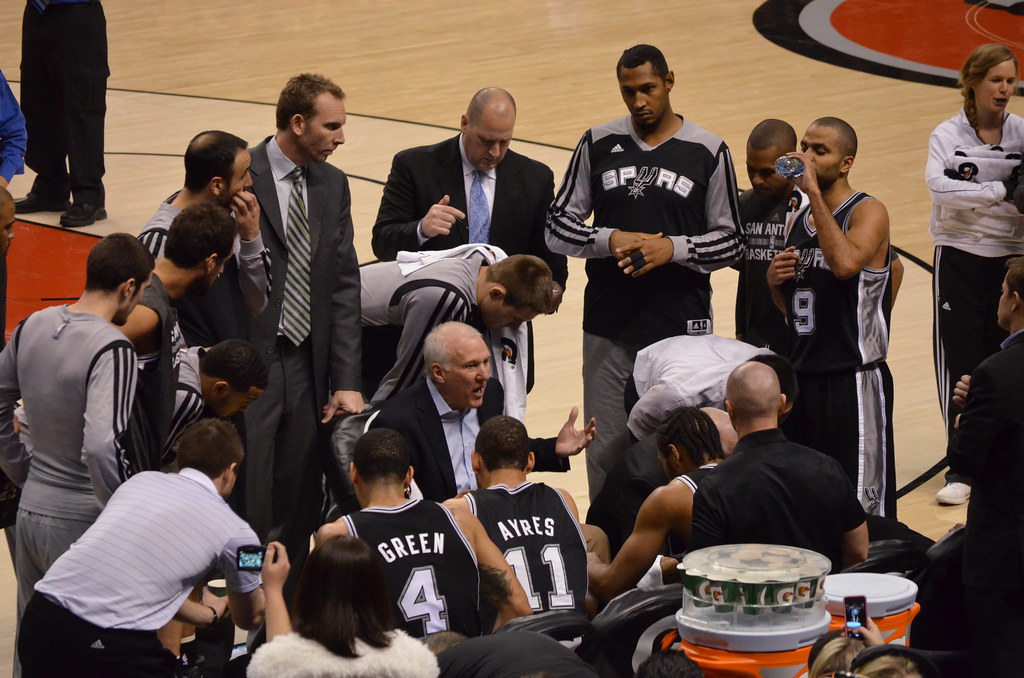In this image, we see a detailed scene of a basketball team from the Spurs gathered for a discussion near the side of the court. The setting is a gym with a light-colored wooden floor featuring accents in red, black, and gray. The focus is on a man with white, sparse hair, seated in a dark-colored suit jacket and a light blue button-up collared shirt, gesturing with his hand as he speaks. This man, presumably a coach, appears to be delivering a pep talk or strategic advice. Surrounding him are several players in black jerseys with white numbers and names; notable players include number 4, Green, and number 11, Ayers. Among these figures, there are other men in sport coats and ties. The players and other individuals are intently focused on the coach, with some seated near him and others standing behind. Additionally, the presence of a Gatorade container filled with cups is visible near the bottom right corner of the image, reinforcing the team's preparation for the game. In the background, parts of the basketball court and an official’s legs can be seen, adding context to the scene's placement in a timeout or team briefing session.